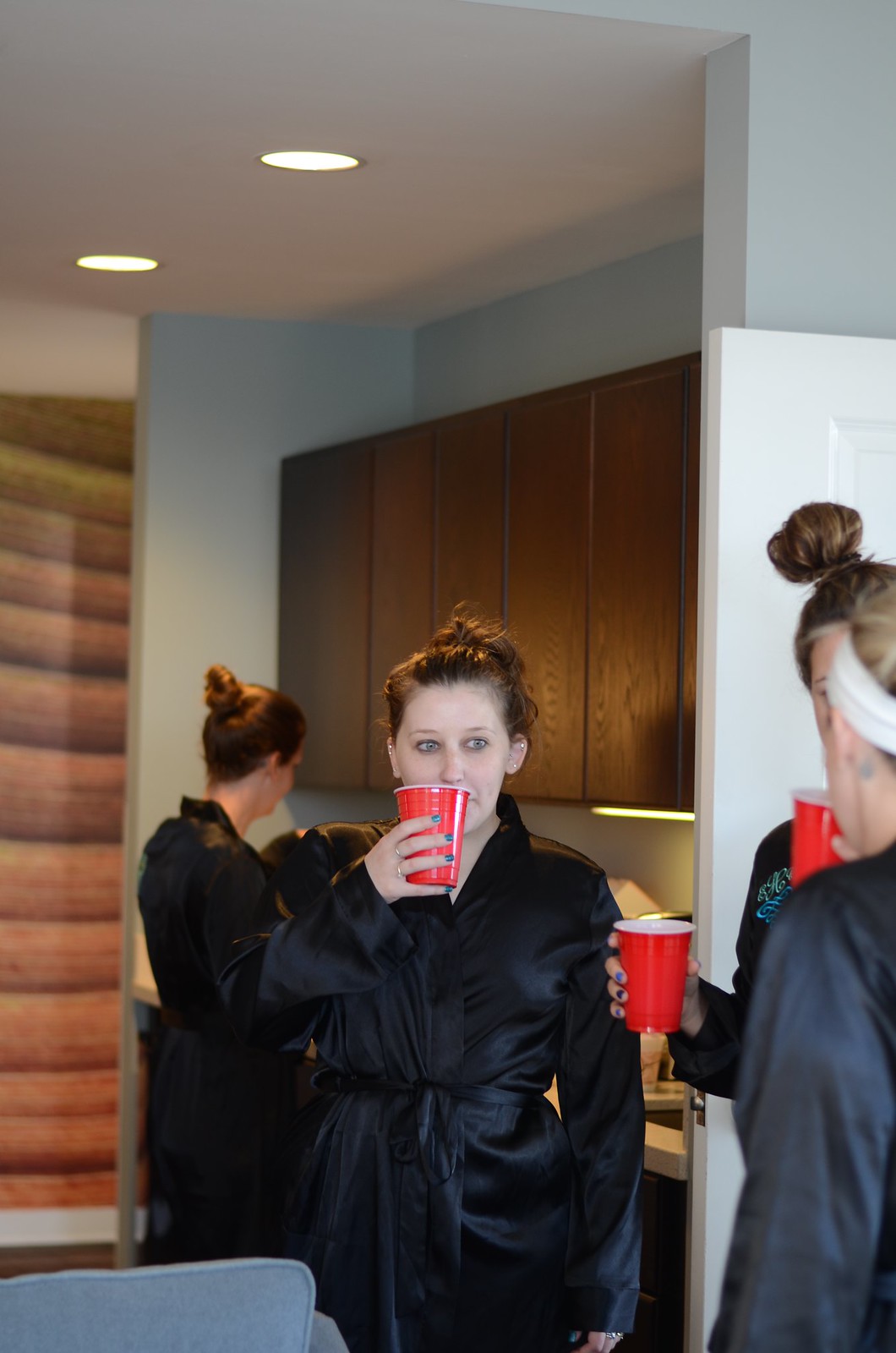In this image, four women dressed in matching black silk bathrobes are gathered in what appears to be a hotel room with dark gray walls and dark brown cabinetry. Three of the women are positioned in the foreground, each holding a red solo cup, possibly containing a beverage. The central woman in the foreground has her hair styled in a messy bun and is captured mid-sip with the cup obscuring her mouth. She gazes off to the right of the frame, not facing the camera. The women on either side of her are only partially visible; one shows just her left ear, while the other, whose hairstyle mirrors the central woman's bun, reveals only her right eyebrow and some hair. All the women have light brown or blondish hair. In the background, near the cabinets and a small countertop, another woman with a similar bun hairstyle is seen, her attention focused away from the group. Spotlights illuminate the dark cabinets, and a bluish-gray chair or object is slightly visible in the lower left of the image. The ambiance suggests they might be preparing for an event, perhaps getting hair or makeup done, under the soft under-lighting of the cabinets. Light blue nail polish can be seen on two of the women, adding a touch of color to the scene.